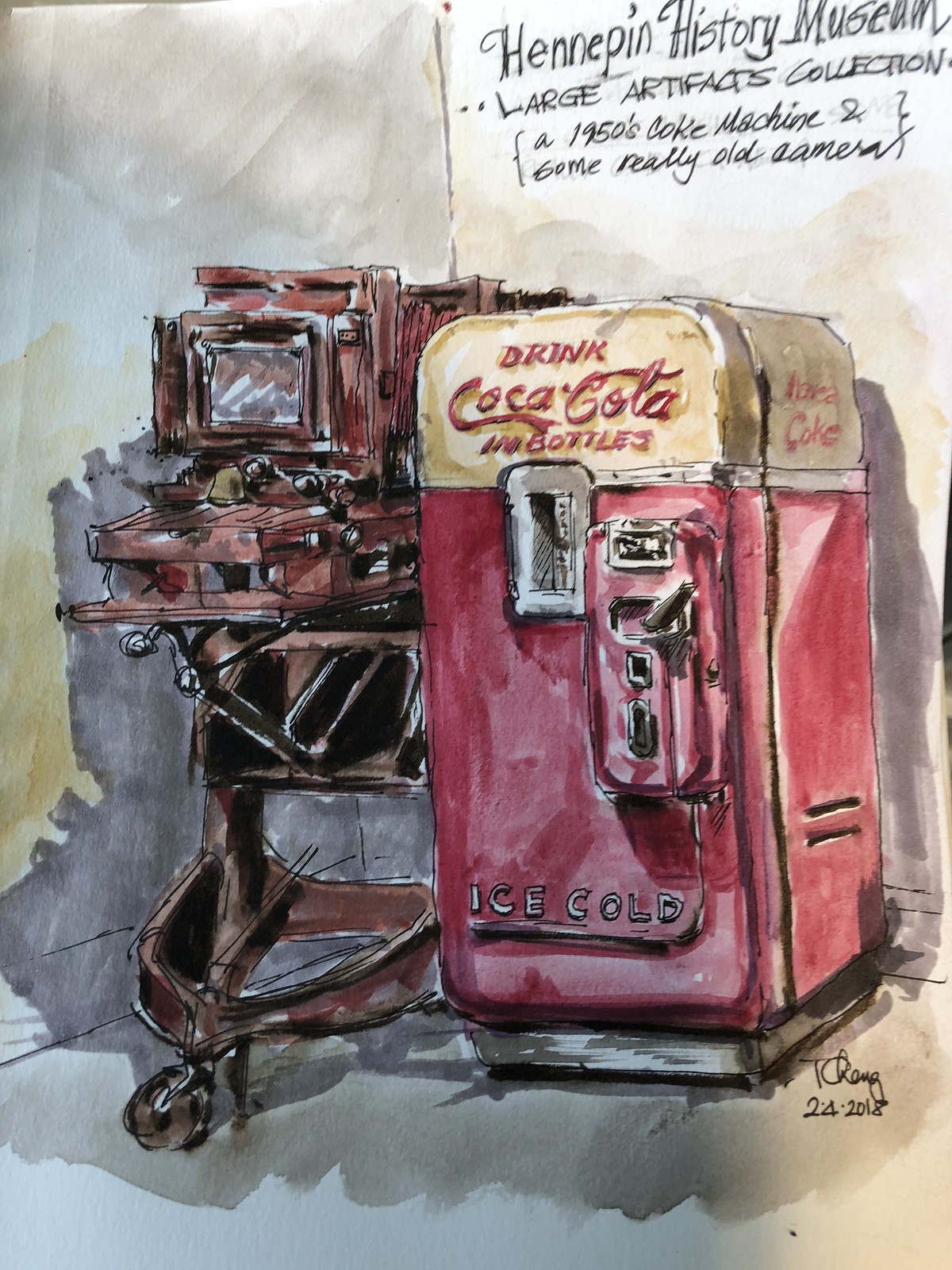This watercolor artwork depicts a nostalgic scene featuring a vintage Coca-Cola vending machine. The machine, boldly painted in classic red and white hues, proudly displays the iconic slogan, "Drink Coca-Cola in Bottles," alongside the phrase "Ice Cold" in striking red lettering. Positioned in a museum setting, identified as the Hennepin History Museum, the artwork showcases the 1950s Coke machine as a central artifact. Adjacent to the vending machine, the painting includes an antique object, which upon closer inspection, appears to be an old-fashioned camera. This intricate watercolor piece captures a moment in history through the lens of these timeless artifacts.